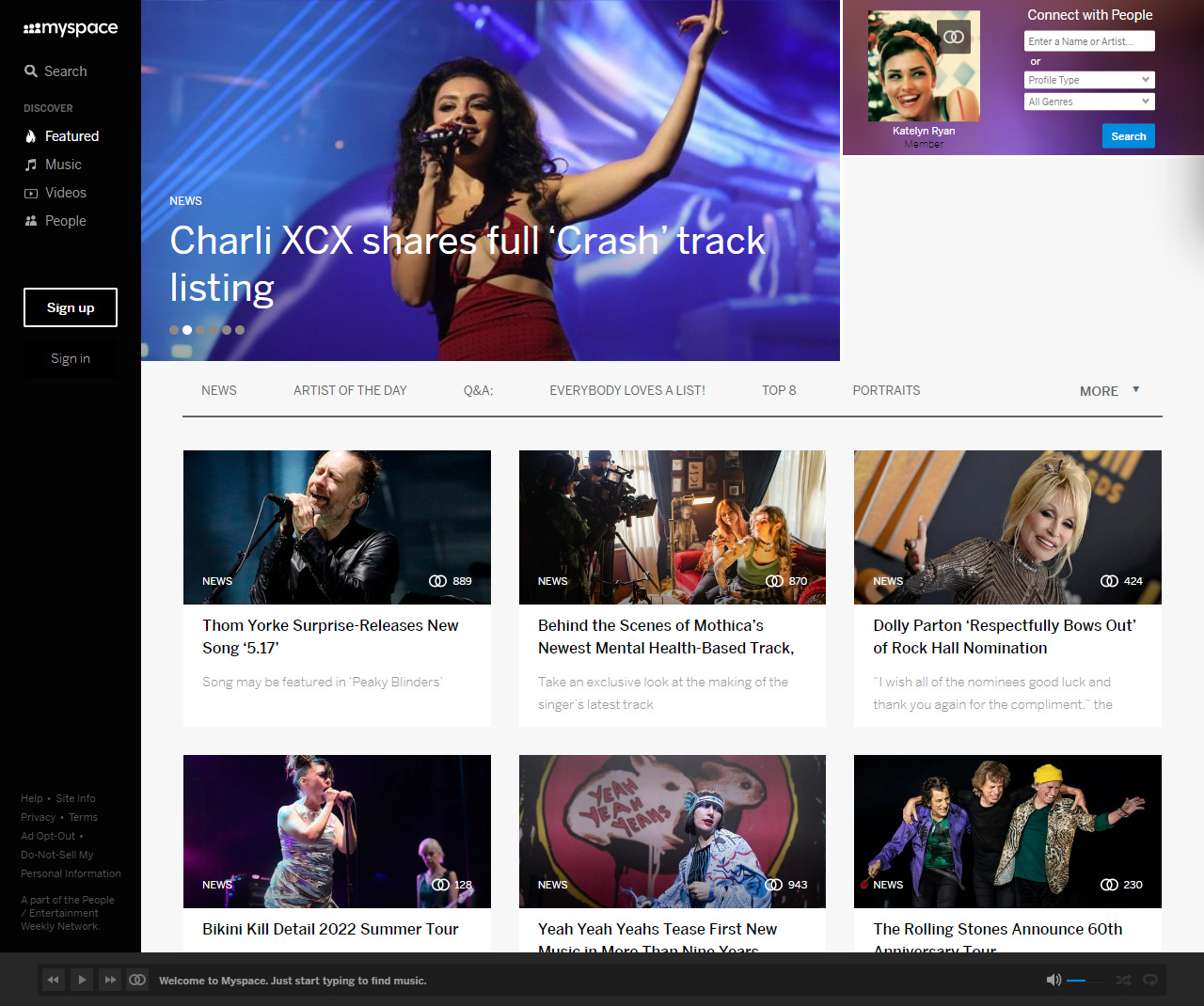This screenshot from MySpace features a black vertical menu bar on the left, with the white MySpace logo prominently displayed at the top. Below the logo is a search bar with a magnifying glass icon, followed by various sections listed vertically:

1. **Discover** (with a flame logo)
2. **Music** (with a note logo)
3. **Videos** (with a YouTube-like logo)
4. **People** (with an icon of two humans)

Below these sections are the "Sign Up" and "Sign In" buttons.

The header of the page highlights a news article: "Charli XCX Shares Full Crash Track Listing," showing Charli XCX performing in concert. The image captures her singing on stage with a microphone in her hand, wearing a red dress against a purple background. This news article falls under the "News" section.

In the upper right corner, there's a prompt to "Connect with People," featuring a thumbnail of a user, possibly named Caitlin Ryan. Users are invited to enter a name or artist and can use a dropdown menu to select "Profile Type" or search across "All Genres."

The menu below the header includes additional sections such as:
- **News**
- **Artists of the Day**
- **Q&A**
- **Everybody Loves Artists**
- **Everybody Loves a List**
- **Top Eight Portraits**
- **More**

Following this, there are six highlighted news items, each accompanied by a landscape photo icon:
1. **Thom Yorke** surprises fans with a new song release.
2. **Behind the Scenes** of Mothica's newest mental health-themed track.
3. **Jolly Partner** respectfully bows out of Rock Hall nomination.
4. **Bikini Kill** details their 2022 tour.
5. **Yeah Yeah Yeahs** tease their first new music in over nine years.
6. **The Rolling Stones** announce their 60th anniversary tour.

Overall, the screenshot effectively captures the diverse offerings and news updates available on MySpace, spotlighting both popular and emerging music artists and events.